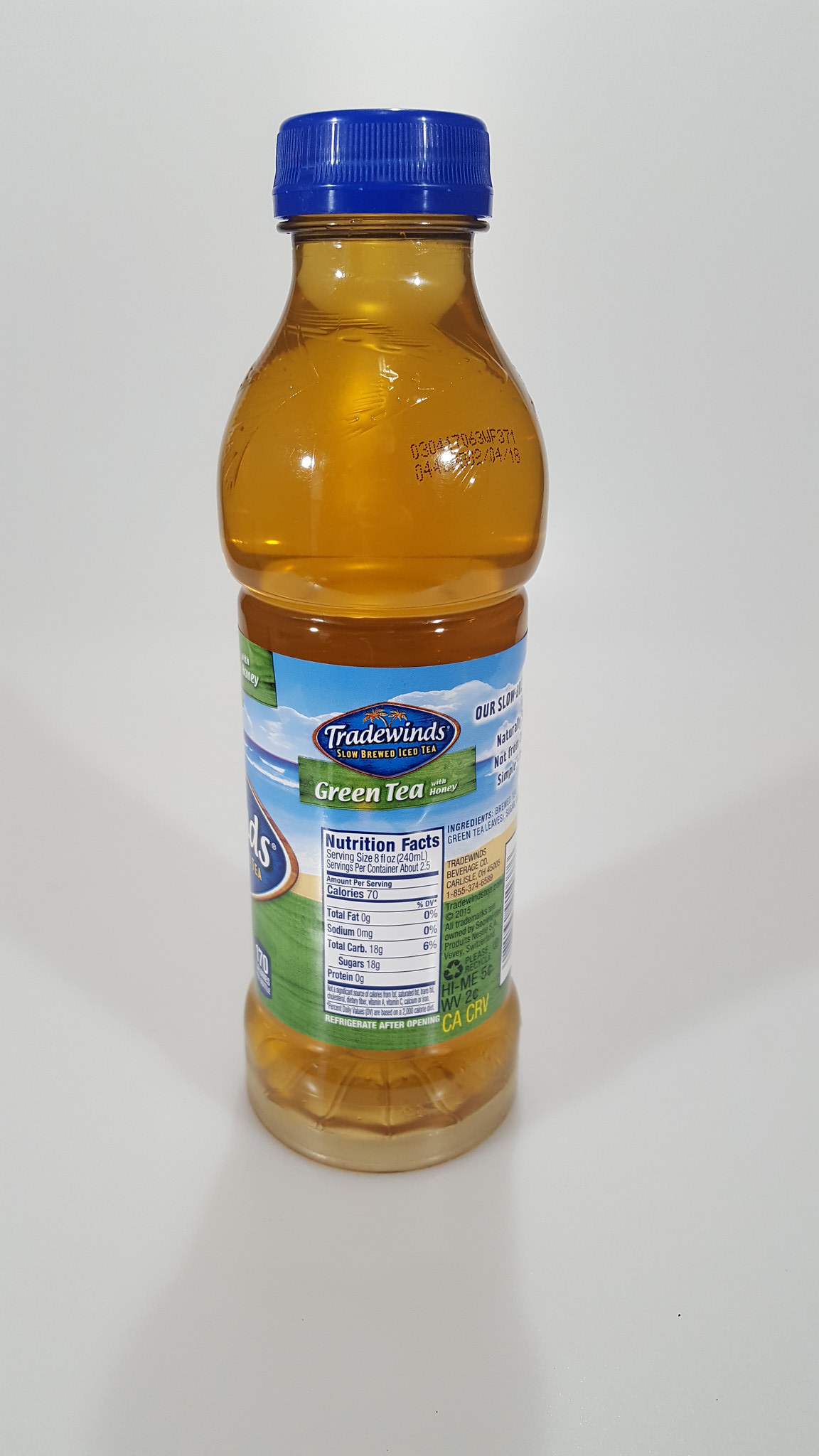This photograph showcases a plastic bottle filled to the brim with a brownish-tan liquid, resembling the color of honey. The label on the bottle reveals that it contains green tea. The label itself features a harmonious palette of blues and greens. Prominently displayed on the label is a rounded diamond-shaped brand logo with the name "Tradewinds" written in white letters. Beneath the logo, within a green rectangular box, "Green Tea" is printed in white text. Below this, another rectangular section contains the nutrition facts, presented in dark blue text. The bottle is topped with a dark blue cap, complementing the overall design.

In the background, a picturesque lake is visible under a bright blue sky dotted with clouds, adding a serene and refreshing context to the scene. The vibrant and natural backdrop juxtaposes nicely with the white surface against which the bottle is placed, creating an appealing contrast that highlights the details and colors of both the bottle and its surroundings.